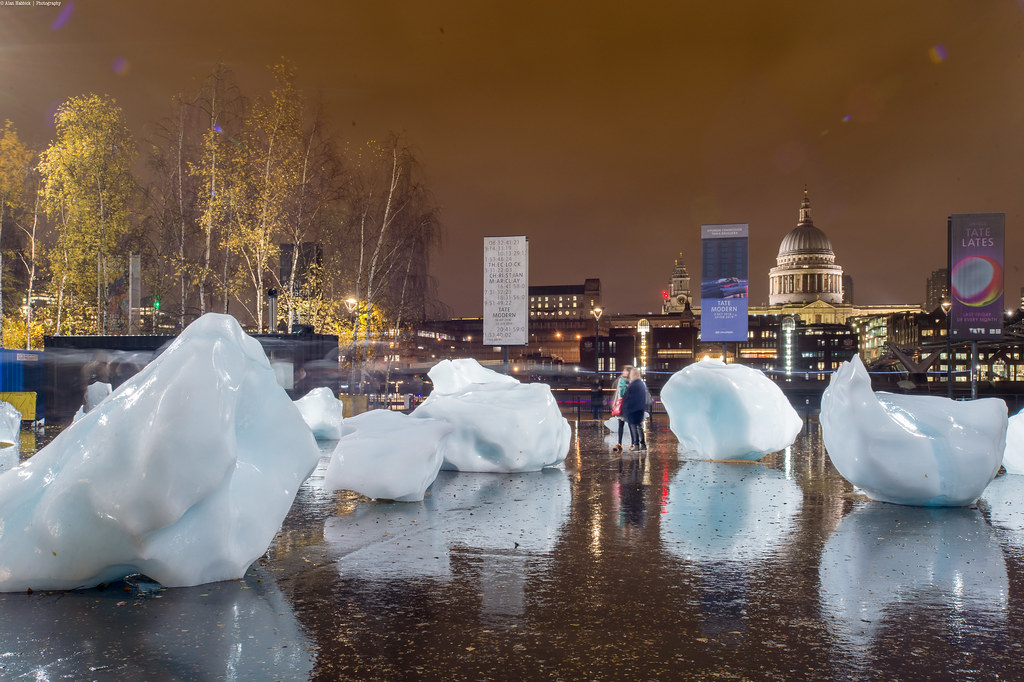The image depicts a dark and rainy scene, likely set in Washington, D.C., featuring a striking arrangement of large ice sculptures resembling icebergs on a wet concrete area. The sky is tinged with a dark brown-orange hue, suggesting late afternoon or early night. Two people stand near these towering ice sculptures, emphasizing their immense size. In the backdrop, tall business buildings, possibly a parking garage, and the Capitol building are visible, illuminated with numerous lights. The wet ground is strewn with fallen leaves. A prominent sign to the right reads "Tate Lates," adding a touch of urban context to the scene.